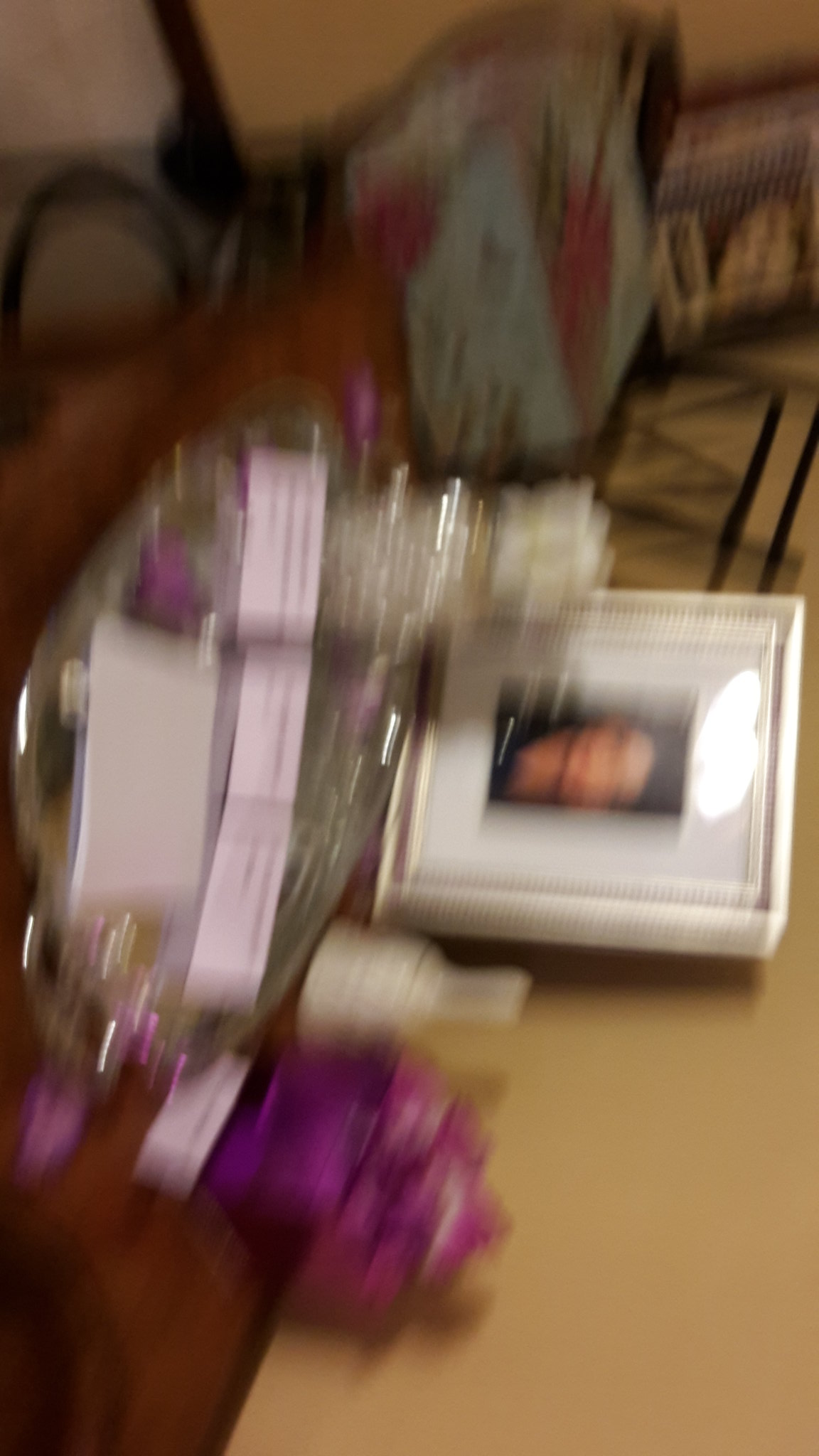This is a very, very blurry photograph taken at an awkward side angle, possibly accidental. The main focus seems to be a small brown wooden table or desk, positioned against a tan-colored wall. Atop this table, there's a framed photo of a woman, which is laying on its back and contributing to the overall blurriness. An overhead light, possibly a ceiling light, adds a white reflection at the top of the image. Scattered around the table are rectangular white cards and various purple items, potentially including a box and a tray. There's also a blank notebook placed at an angle on the table's edge. Colors in the scene include pink, fuchsia, terracotta, white, beige, and black, though they are all melding together due to the poor focus. The chaotic arrangement and reflections make it difficult to discern individual items clearly.